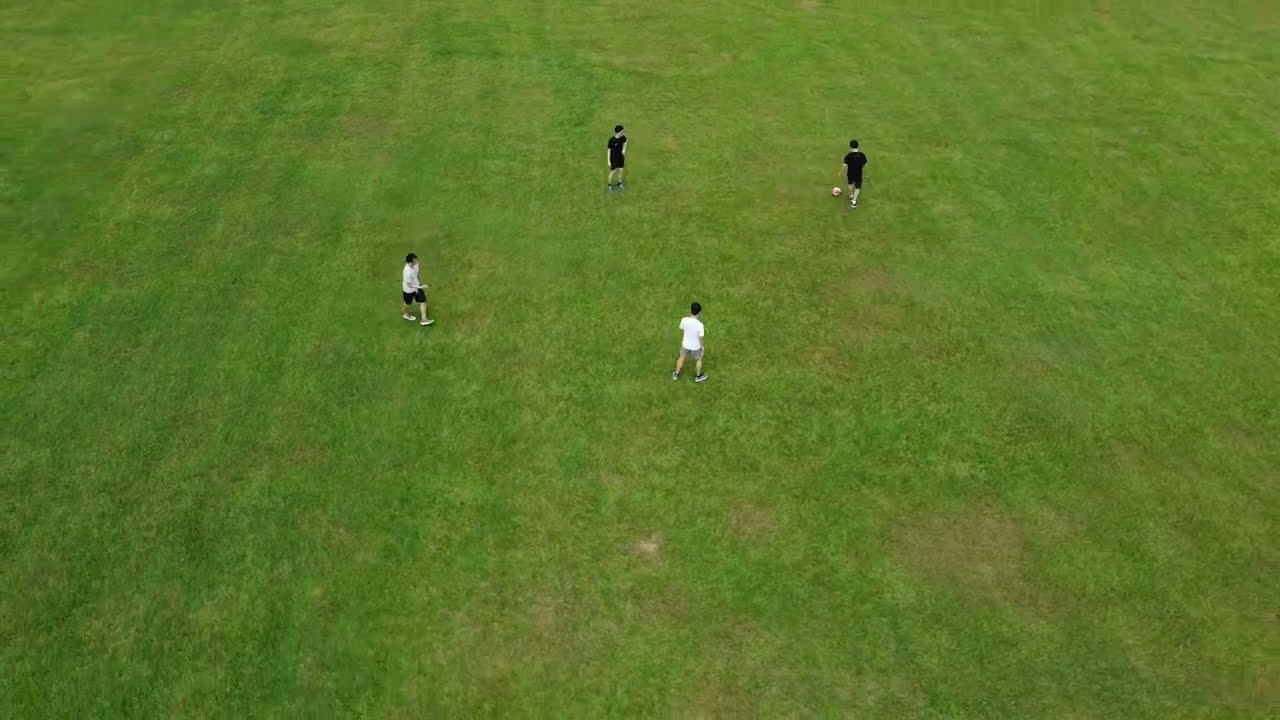The image captures a recently mowed, lush green field with visible mowing stripes. Four young men are positioned in a square-like pattern on the grass, with two wearing white shirts and the other two in black shirts. The individual in the upper right corner, dressed in black, is about to kick a soccer ball while the remaining three—two in white below and slightly left, and the other in black above them—are attentively watching. The field is devoid of any visible goals or painted lines, suggesting the game may be informal or the goals are out of the camera’s range. The scene looks casual, possibly a practice session or a friendly game, with the players engaged in what appears to be either a game or just kicking the ball around. The well-kept grass field has some brown spots scattered throughout, adding a touch of realism to the scene.